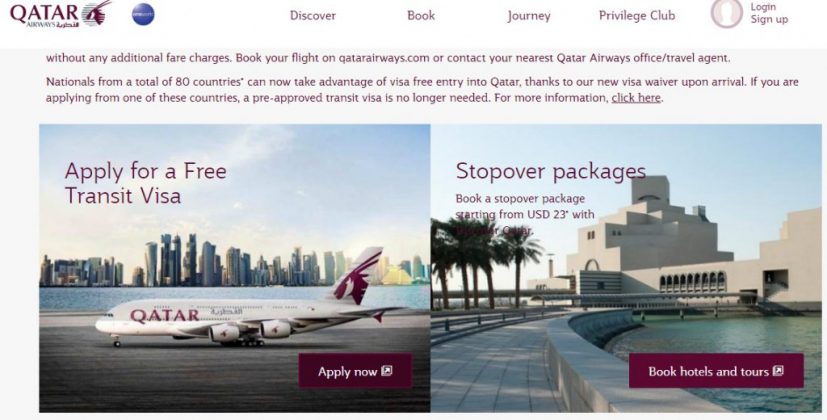**Descriptive Caption: Qatar Airways Web Page**

At the top left of the Qatar Airways web page, the airline's name "QATAR" is prominently displayed in maroon red, accompanied by an animal symbol, likely reflecting the brand logo. The top right features a navigation bar with tabs labeled: "Discover," "Book," "Journey," "Privilege Club," "Log In," and "Sign Up."

The main section of the page has a dark grey background with eye-catching red text at the top. On the left side, a striking image of a Qatar Airways airplane shows the word "QATAR" in large maroon letters on the fuselage and the animal logo on the tail wing. Below the image, a maroon rectangle button with white text invites users to "Apply Now."

Adjacent to this, a small graphic overlay features a square with another square on top of it and an arrow pointing to the right. Above this, in maroon text, it says, "Apply for Free Transit Visa." In the background, a cityscape reminiscent of New York City is visible, with cyan blue water and a sky dotted with white clouds.

On the right side of the page, a prominent dark grey building with a matching path leading to it is showcased. Above this, the text "Stopover Packages" is inscribed, advertising stopover packages starting from USD 23. Below this section, a maroon rectangle with white text encourages users to "Book Hotels and Tours," featuring another graphic with a square and an arrow.

The red maroon text at the very top in the dark grey header reads: "Without any additional fare fees. Book your flight on QatarAirways.com or contact your nearest Qatar Airways office or travel agent." It highlights that nationals from 80 countries can now take advantage of visa-free entry into Qatar, thanks to a new visa waiver upon arrival, making pre-approved travel visas unnecessary for these nations. For more information, a hyperlink is provided labeled "click here."